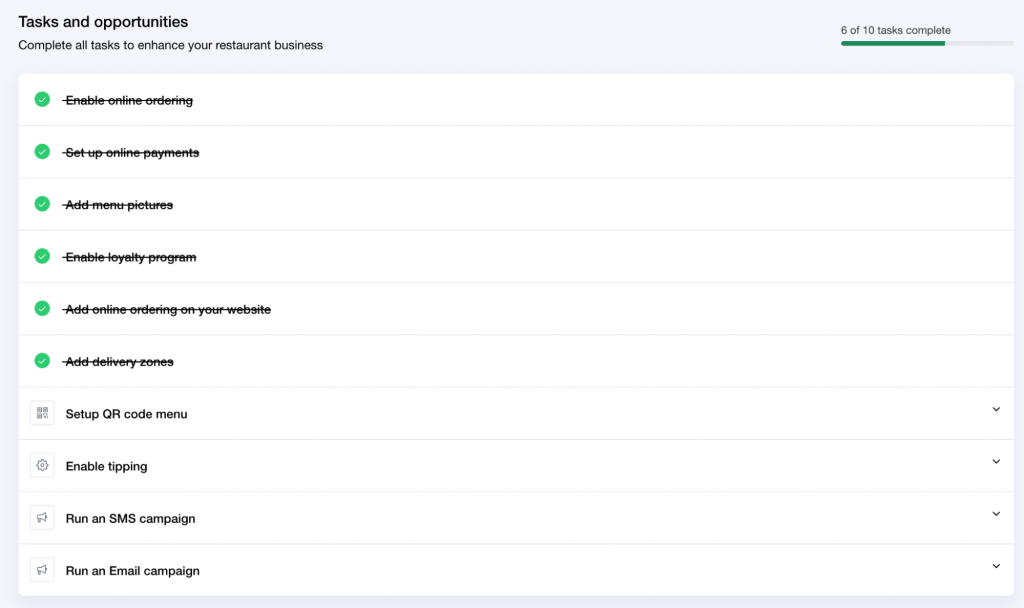The image features a light blue background with a prominent section titled "Tasks and Opportunities." Below this title, there's a message stating, "Complete all tasks to enhance your restaurant business." On the right side of the image, a status indicator reads "6 of 10 tasks complete" alongside a progress bar filled in green. Dominating the center of the image is a large white box containing a list of tasks.

The first six tasks have been completed and are marked with green circles bearing check marks and strike-through lines. These tasks are followed by four additional, incomplete tasks, each accompanied by a downward-pointing arrow. The incomplete tasks are: "Set up QR code menu," "Enable tipping," "Run an SMS campaign," and "Run an email campaign." The entire list, both completed and pending tasks, is set against the same light blue background, encapsulating the focus on task management and opportunities for enhancing the restaurant business.